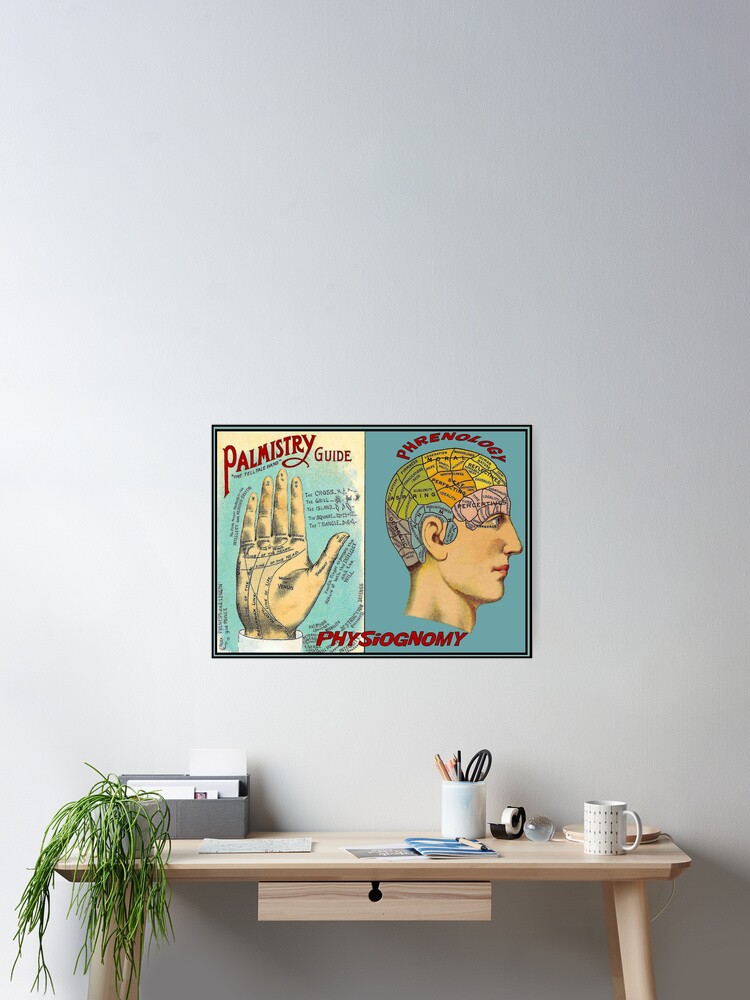This indoor color photograph features a light brown desk positioned in the lower right-hand corner against an off-white wall. The desk, with its blonde wood top and spindle legs, has a single drawer in the middle. On the far left side of the desk is a small green plant with long leaves hanging over the side, and behind it is a gray box likely holding envelopes. In front of this box lies a piece of paper. Moving rightward on the desk, there is a white holder filled with pencils and scissors. Adjacent to it is a roll of scotch tape in a black case, followed by a white coffee mug. In the far right-hand corner stands a white lamp. Directly above the desk, a piece of artwork is displayed. The left side of the artwork features a palm with the label "Palmistry Guide" above it in red letters and annotations in black. The right side showcases a human head with the brain area mapped out in multicolored regions, labeled "Phrenology" above it. Across the bottom of the artwork, it reads "Physiognomy" in red letters.